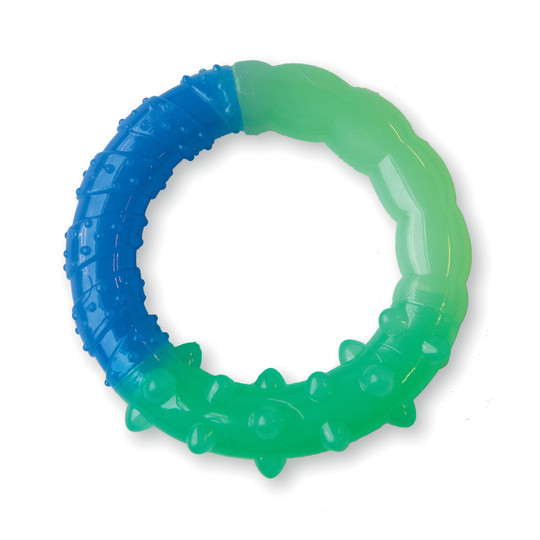The image features a plastic ring teether, displayed on a clean, white background. The ring is divided into two distinct sections: approximately two-thirds of it is a smooth green portion with a lower segment adorned with small spikes. The remaining third is a blue section that has an intricate pattern of stripes and dots, sporting a semi-shiny, slightly rubbery appearance. Both sections come together to form a round, textured ring, hinting at its potential function as either a teething ring or a versatile toy. The photograph does not include any labeling or branding, leaving the exact dimensions and specific purpose of the item open to interpretation.